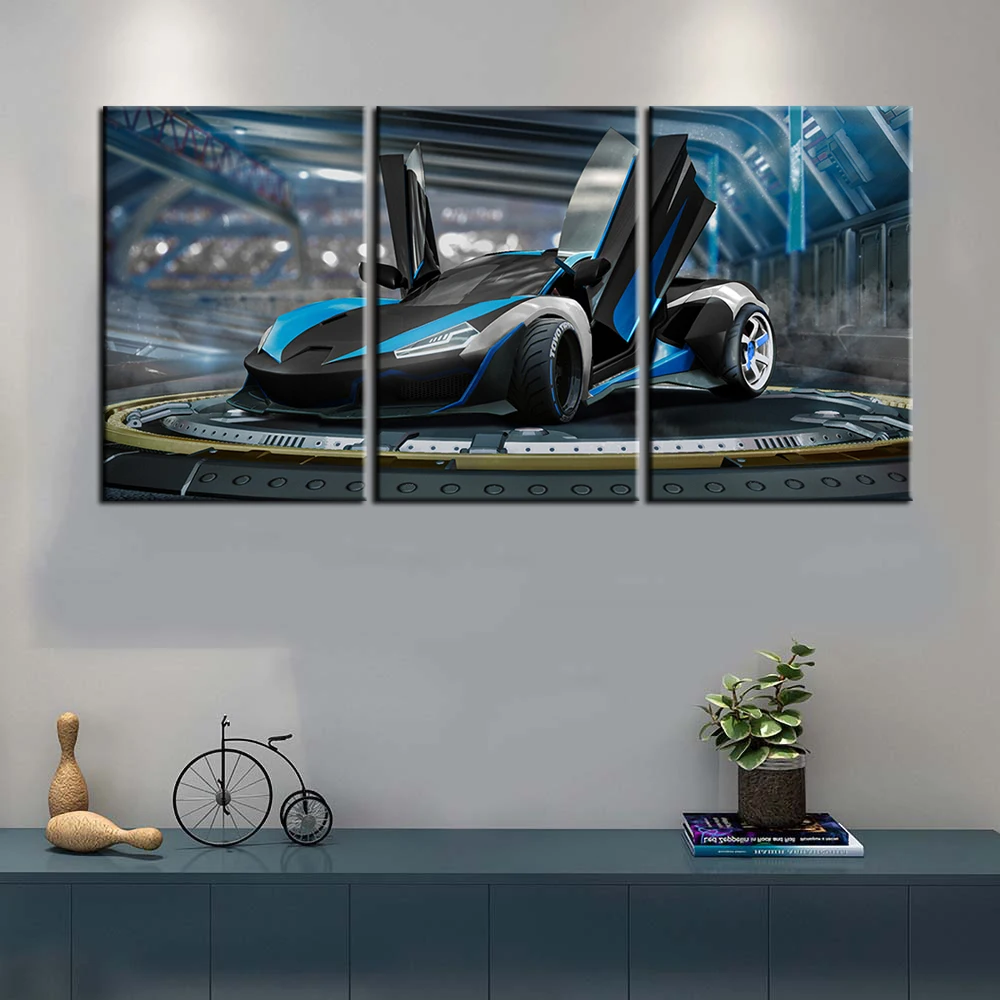This is a detailed color photograph of a stylish domestic living room or entryway, showcasing a sleek, modern setup perfect for product demonstration. Against a pristine white wall, a narrow table or shelf runs along the bottom edge of the image, adorned with various decorative objects including an old-fashioned tricycle model with a large front wheel, two vintage wooden bowling pins, a potted succulent, and some books or magazines.

Dominating the center of the photograph is a striking piece of wall art composed of three canvases, collectively displaying a single cohesive image of a futuristic sports car. The car, predominantly black with vivid blue and silver accents, is shown with its distinctive upward-opening doors resembling bat wings. It appears to be poised on a rotating platform, suggestive of a display at a car show or an indoor futuristic race track. This meticulously arranged scene captures both the elegance of the decor and the high-tech allure of the featured artwork, making it a compelling visual attraction.